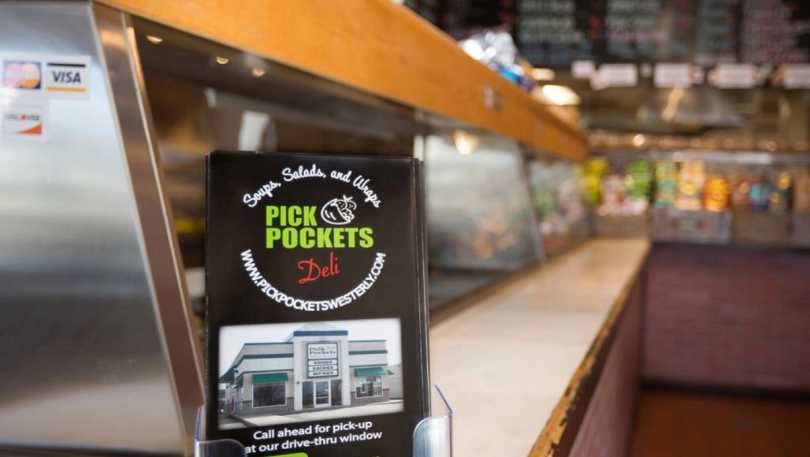This is a detailed photograph of the interior of Pickpockets Deli, viewed from one end of the counter stretching towards the back. The primary focus of the image is a stack of black pamphlets prominently placed near the left side of the counter. These pamphlets, likely menus, feature white lettering at the top stating "Soups, Salads, and Wraps," and in the center, green text reading "Pickpockets," accompanied by a black-and-white logo of a pita pocket. Below this, "Deli" is written in red, followed by the URL "www.pickpocketswesterly.com" and an image of the deli's exterior with green awnings. Additionally, there is a prompt: "Call ahead for pickup at our drive-thru window." The counter itself is accented with light yellow or brown framing, with a metal silver display case adjacent to it, displaying logos for MasterCard, Visa, and Discover. In the background, partially blurred, are food items and a chalkboard menu on the wall.